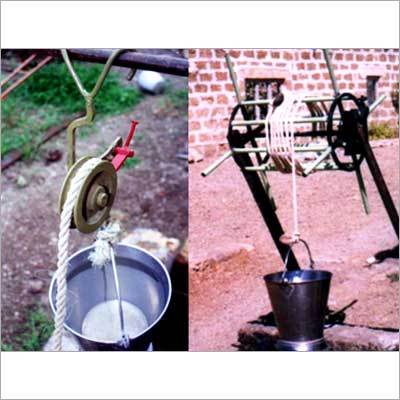In this side-by-side image set, both pictures depict historical pulley systems likely used for wells. On the left, we see a close-up view of a pulley system featuring a copper-colored pulley positioned in the center of the image, attached to a horizontal bar at the top. A white rope runs over the pulley, connected to a silver bucket that appears filled with water, situated in the lower third of the image. The background showcases green grass beneath the bucket with a bisecting trail on the left. On the right, a more complex pulley setup is presented. This system includes two wheels connected by horizontal bars around which a rope is wrapped multiple times. The pulley is constructed from black metal, and a darker gray bucket hangs at the bottom center. The background consists of red-brown dirt and a red brick building featuring a couple of windows in the upper third of the image. Both images, grainy and old-looking, highlight different yet functionally similar well pulley designs used for raising and lowering buckets.